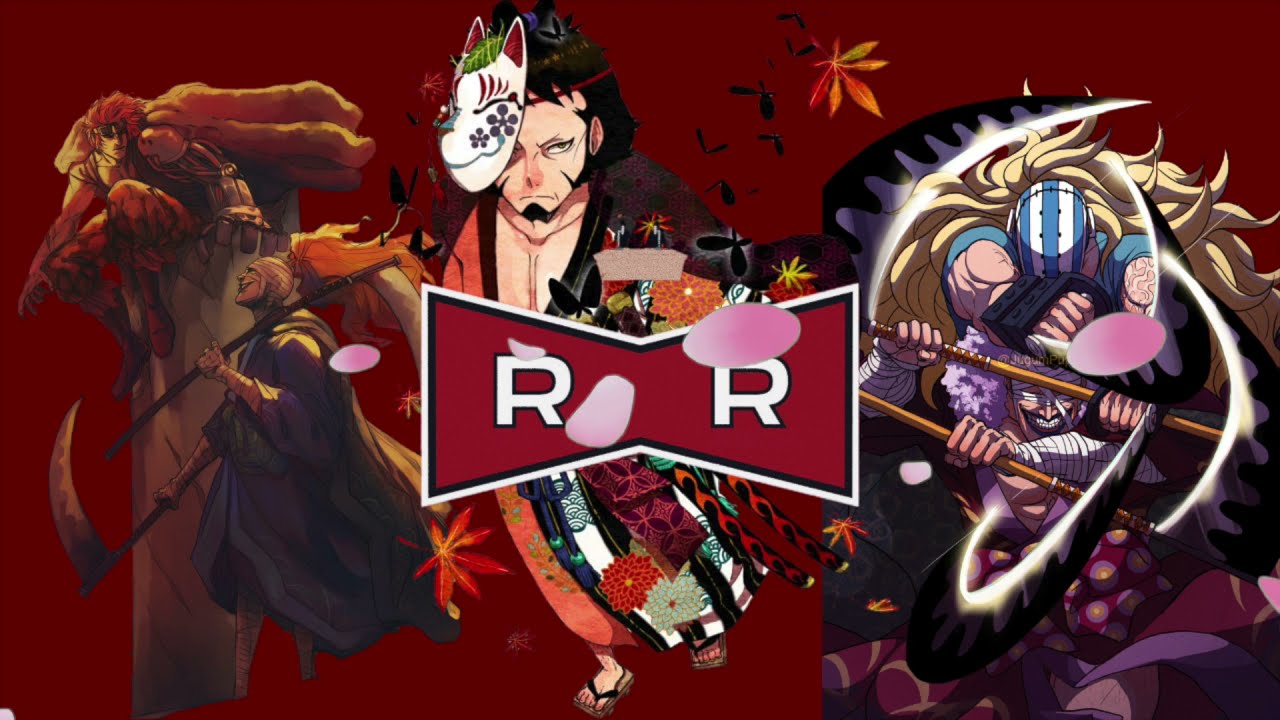This animated image, possibly designed for a video game, is set against a dark maroon background and features four distinct characters in detailed, anime-style illustrations. On the far left is an orange-hued, smoke-like entity with an oversized body and a small head adorned with four indistinct arms. Next to it stands a figure resembling a grim reaper, the smallest in stature, clad in a dark cape from neck to toe and wielding a scythe and a spear. This character is notably distinguished by a Roman soldier helmet with a gold feather. 

At the center of the composition, in front of a horizontally oriented, red bow-tie shaped logo inscribed with the letters "RR," is a samurai-like figure. This central character dons a colorful, long robe and black sandals, with black hair and a cat mask perched partially on the side of his face. He sports a black goatee, adding to the elaborate detail.

The fourth and largest character, positioned on the far right, is somewhat ambiguous but appears to have eyes at the top, possibly wearing a robe, and is associated with a swath of white light. This character is also depicted holding a bow staff. Throughout the background, there are elements such as falling flower petals and birds, adding a dynamic and intricate touch to the maroon and dark red backdrop.